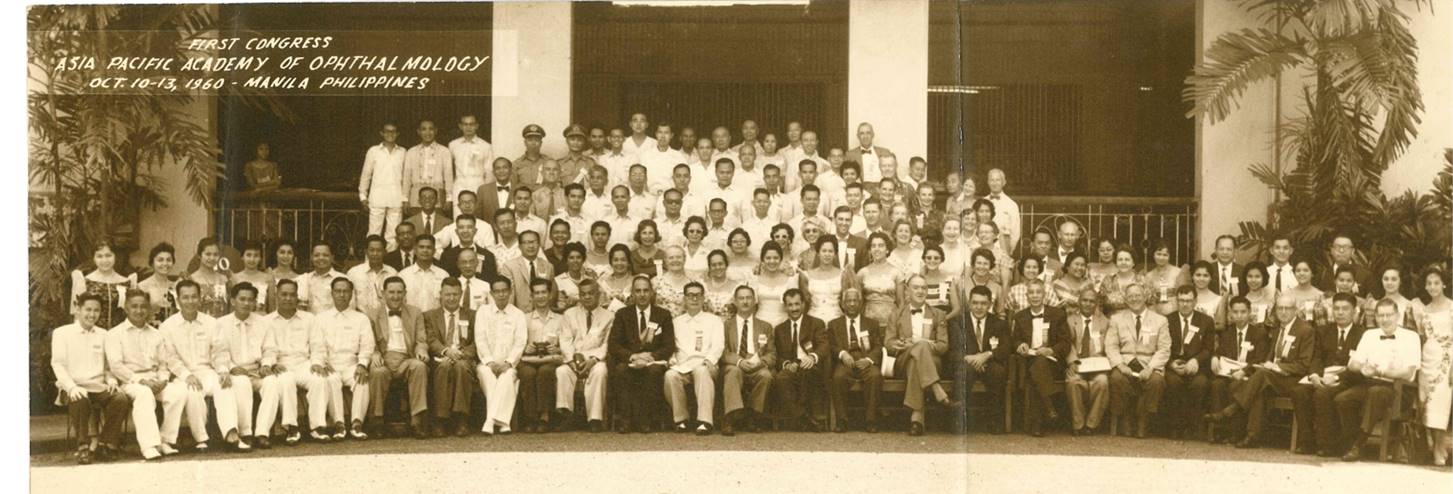This black and white panoramic photo, with aged tones lending it a brownish hue, captures a large assembly of individuals posed in front of a white stucco building adorned with three dark openings, balconies, and flanked by tall palm trees on either side. The photograph bears a watermark in the upper left-hand corner that reads: "First Congress Asia-Pacific Academy of Ophthalmology, October 10-13, 1960, Manila, Philippines." This historic image from the 1960s shows a meticulously arranged group, with the first row of individuals seated and dressed in a mix of white coveralls and traditional black suits. Behind them, up the steps leading to the building, are six or seven additional rows of people, predominantly in white attire. The image shows some signs of aging and damage, adding a textured layer to its historical significance.